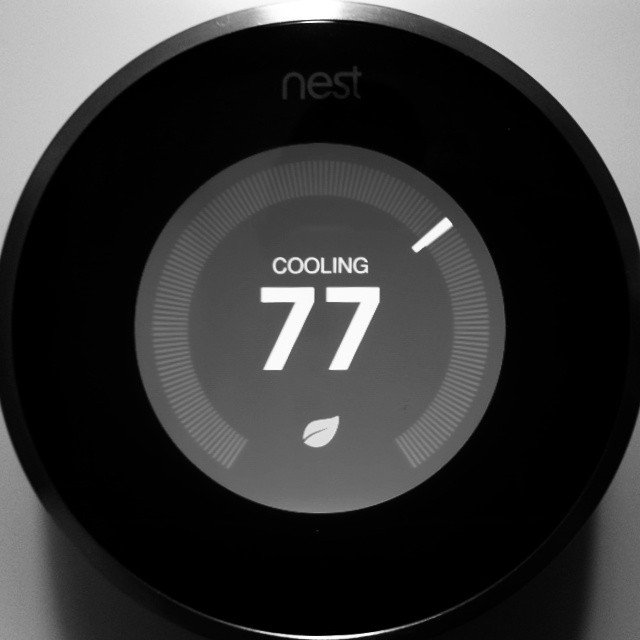This close-up indoor photograph features a Nest thermostat dial prominently displayed against a white wall. The outer ring of the dial showcases a brushed metal finish, while a black ring encircles the dial. At the 12 o'clock position, the brand name "Nest" is clearly visible in white letters. The center of the thermostat displays a gray disc, which contains an array of tiny lines indicating the current thermostat setting. The word "Cooling" is displayed in white letters at the center, along with the current temperature setting of 77 degrees. Additionally, a green eco leaf symbol is present, signifying that the thermostat is in eco mode. The white wall background is subtly visible in each of the four corners of the image, further highlighting the sleek design of the thermostat.